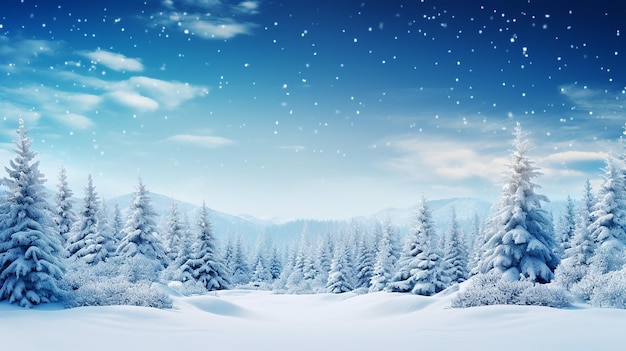This image, which appears to be created with a smooth, slightly edited style—possibly drawn, painted, or computer-generated—captures a serene winter outdoor scene in the mountains. The horizontal rectangular frame depicts a dark blue to light blue gradient sky, dotted with white clouds and softly falling snowflakes, lending a dreamy, somewhat fuzzy atmosphere. In the distant background, the haze-shrouded black mountains are capped with white snow. Dominating the middle of the scene, a dense forest of tall pine trees, laden with snow, stretches from one side of the image to the other. The foreground features a pristine, rolling snow-covered field, with occasional bushes or plants blanketed in snow. There are no humans or text present, allowing the landscape's tranquil, snow-laden beauty to shine through.